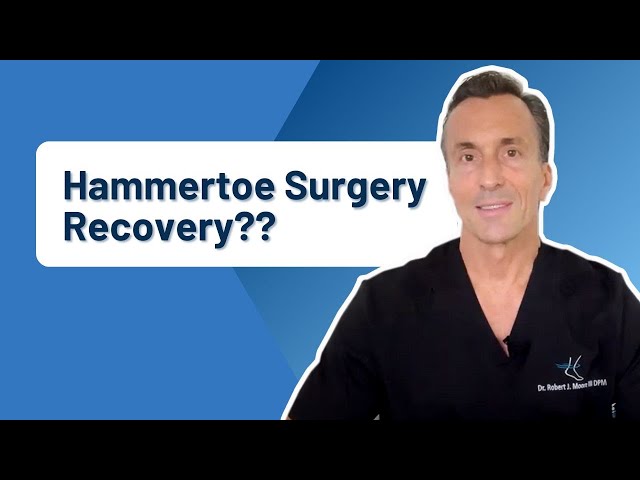The image features a polished advertisement for a doctor, likely intended for digital media such as a website banner or a video thumbnail. Encased by black borders at the top and bottom, the central section showcases a doctor against a blue background with a geometric pattern in varying shades of blue. On the right side of the image, prominently outlined in white, is Dr. Robert J. Moore III, DPM. He is a Caucasian man with neatly parted short brown hair, brown eyes, and a confident, reassuring smile. He wears hospital scrubs, and on the right side of his chest, there is an embroidered insignia of a foot with a blue line around the ankle, reflecting his medical specialty. Next to him, extending into the middle of the ad, is a large white text box with bold navy blue lettering that reads, "Hammertoe Surgery Recovery???"